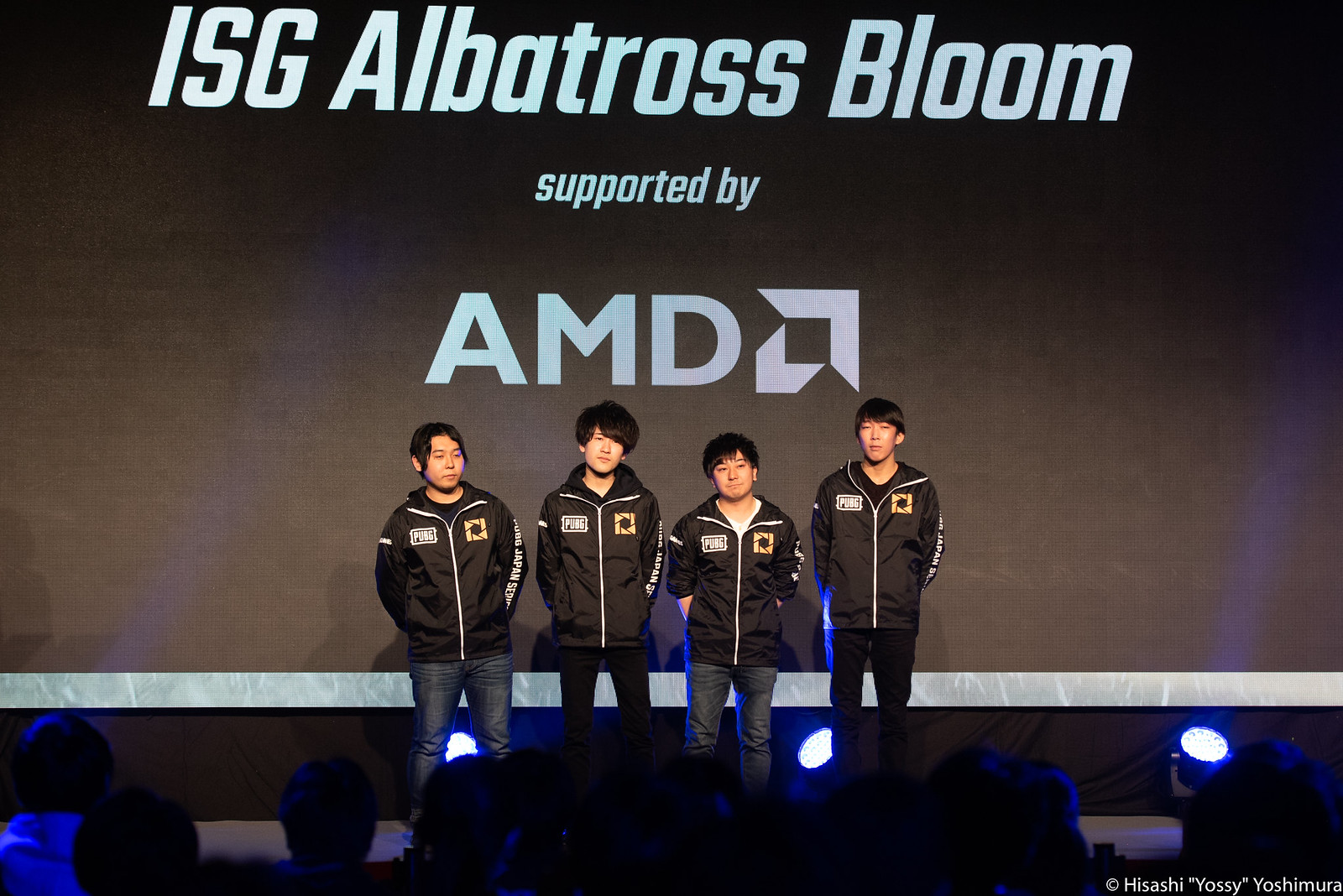This image captures a team of four young Asian men, likely in their late teens to early 20s, attending an eSports event. They're standing on a stage, all wearing identical black jackets with white zippers and white detailing. The jackets feature a yellow or gold emblem on the upper left side pocket, and the words “PUBG Japan Series” run down the sleeves, indicating their association with the popular video game. Behind them is a brightly lit projection screen that reads "ISG Albatross Bloom, supported by AMD." The photo seems to be taken at a press event or convention, with an audience visible in the foreground, suggesting a large gathering. Each team member has a serious expression, with their hands either in their pockets or behind their backs, exuding a professional yet composed demeanor.